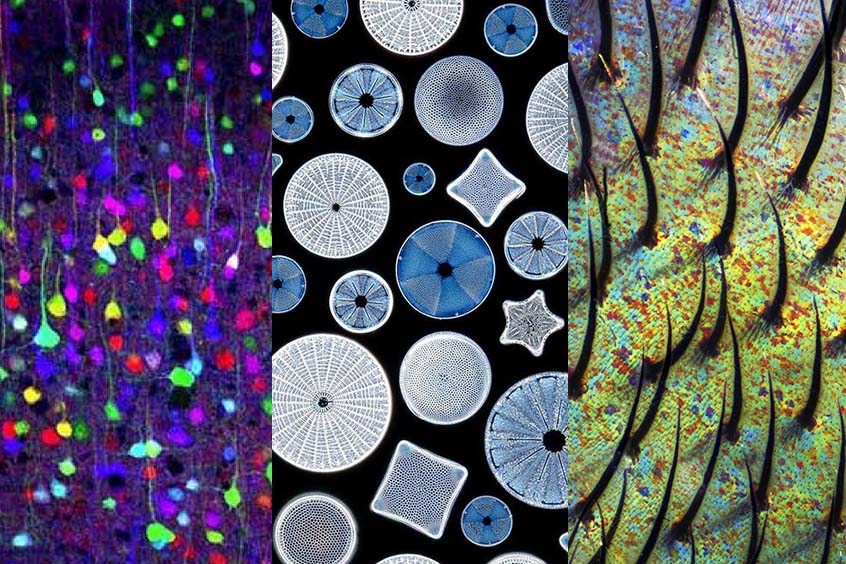This image is a modern art piece divided into three distinct sections, all housed within a horizontally elongated frame. The left section features a dark purplish background adorned with a myriad of brightly colored shapes in reds, yellows, greens, and blues. This part evokes the image of passing through a beaded curtain, with the hues and patterns creating a vibrant and somewhat transparent effect.

In the middle section, against a stark black background, are a variety of circles in different sizes and colors, predominantly blues and grays. Some circles exhibit intricate patterns, resembling spokes in white and light blue, while others have random, non-repeating shapes. This section also includes tilted squares with white borders, surrounded by an array of smaller and larger circular forms, creating a complex, wallpaper-like design.

The right section appears as a highly magnified image of hair follicles sprouting from a multicolored surface. The background blends oranges, reds, light blues, and purples, with dominant orange and red tones. The "hair" structures are sparsely spaced, resembling thorns or spikes, set against this mottled, skin-like texture. The upper left corner of this section shifts toward bluish and purplish hues, adding to the surreal and otherworldly quality of the overall piece.